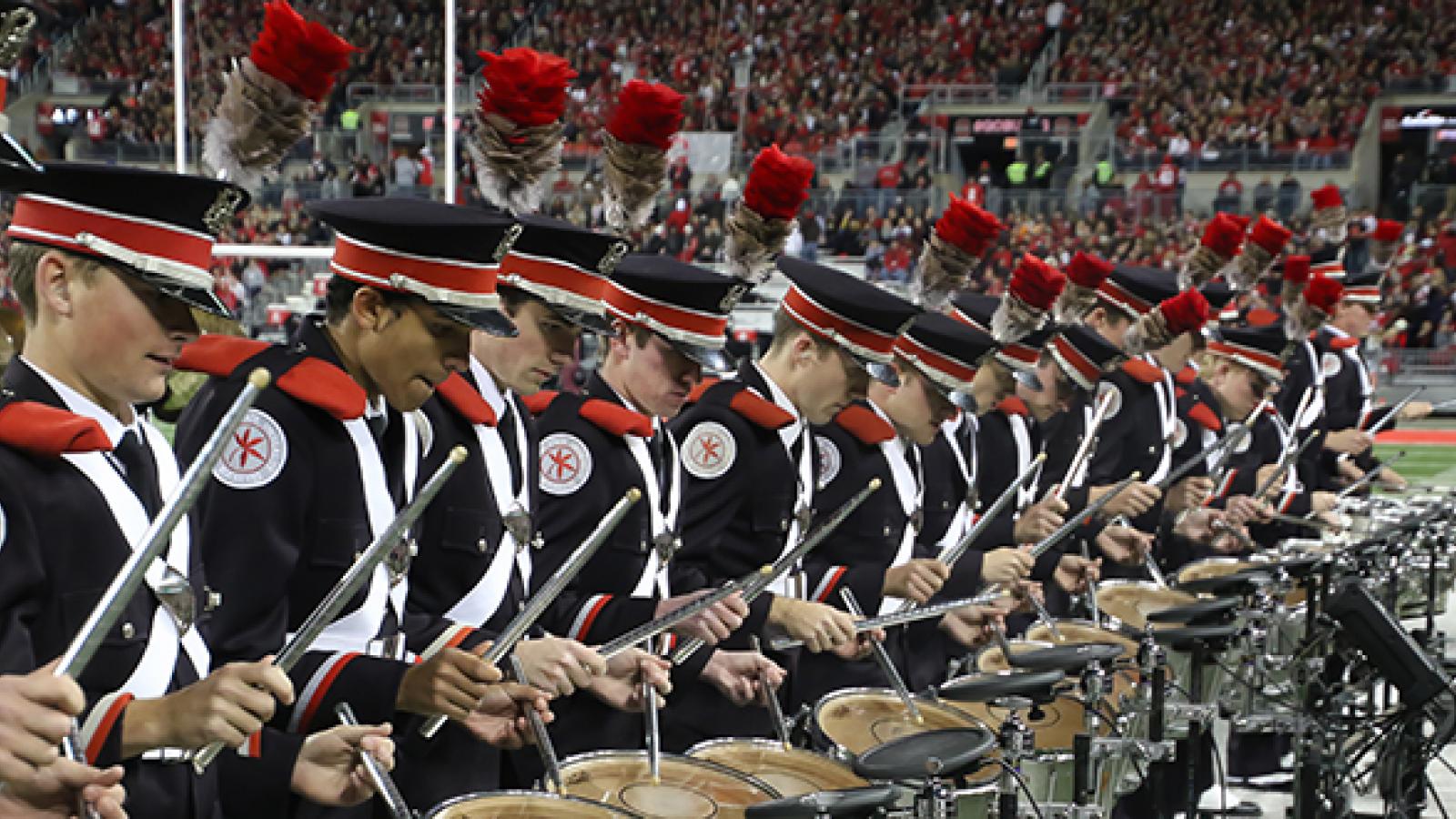In this horizontally oriented, realistic photograph taken at a football game in an outdoor stadium, a snare drum line is featured prominently in the foreground. The drummers, all men, are lined up shoulder to shoulder, each holding silver drumsticks and playing with a dual grip position. They wear matching black uniforms accented with blue suit jackets, white X sashes across their shoulders, blue ties, and white shirts. Their hats are black with a red band and a red and white trim. The stadium is filled with a large crowd, predominantly dressed in red, giving a vibrant and intense backdrop. A white goalpost is visible in the back left, and some unreadable text is faintly seen on the football signs. The drummers are intensely focused on their performance, creating a captivating sight as they play in unison.